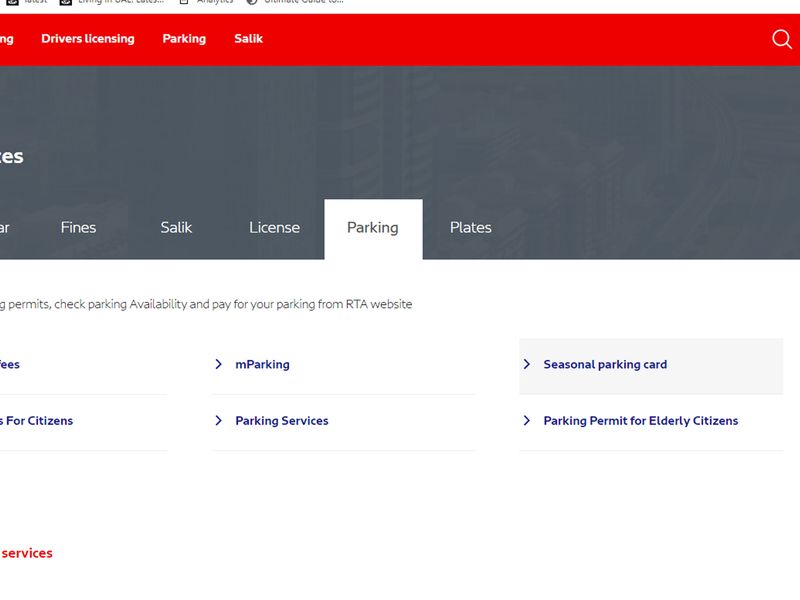**Screenshot of Parking Website Interface**

This screenshot captures a partial view of a parking-related website. The image showcases the top right corner of the webpage, highlighting several distinct areas and features.

At the top, there is a prominent red header. The first word in the header is partially obscured, displaying only the letters "NG." Within the header, there are various navigation options in white text, including "Driver's Licensing," "Parking," and "SAILIC." To the far right of the header, a white magnifying glass icon represents the search function.

Below the red header is a dark gray section occupying approximately half of the visible screen. This section also contains partially visible text starting with the letters "ES." Beneath this text lie a series of selectable options. From left to right, these options read: "AR" (partially cut off), "Fines," "SAILIC," "License," and "Parking." The "Parking" option is highlighted with a white rectangle and gray text, indicating it is the currently selected page. Adjacent to these, there is an unselected option labeled "Plates" against the dark gray background.

The lower half of the screenshot features a white background with additional content fragments. Visible text includes the letter "G" followed by "permits," with a subheading that reads: "Check parking availability and pay for your parking from RTA website." Below this, there are several dropdown options in blue text, though some are partially visible. These options appear to be titled "Fees" (displaying as "EES"), "S for Citizens," "M, parking," "Parking Services," "Seasonal Parking Card," and "Parking Permit for Elderly Citizens."

This detailed screenshot provides a glimpse into the navigation structure and some functionalities available on the website.